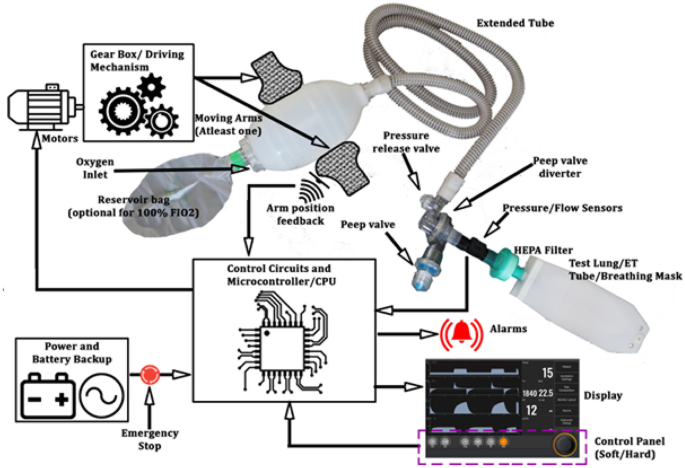This detailed diagram illustrates a complex filtering or respiratory system, featuring an interconnected network of components. Starting in the upper left corner, a small device plugs into a labeled gearbox driving mechanism, depicting three black and white wheels. Adjacent to the gearbox on the right is a box tagged control circuits and microcontroller, inclusive of a CPU. Below, in the lower left, resides a box showing a battery with positive and negative signs, labeled power and battery backup, with a circle and squiggly line above it. An arrow from here directs to the control circuits.

Further right, another arrow points to an alarms section showcasing a red bell icon between parentheses. The lower right corner of the diagram features a black display box with digital numbers, titled display control panel, with "soft/hard" in parentheses. Above this, a white handle with a green attachment and an upward-extending hose is labeled as the extended tube.

Additional arrows and labels denote multiple components surrounding these main sections, such as the pressure release valve, PEEP valve diverter, pressure flow sensors, HEPA filter, oxygen inlet, motors, reservoir bag for 100% FiO2, test lung with ET tube, and a breathing mask.

This diagram provides a meticulous breakdown of a mechanical system, possibly related to a respiratory aid or filtration unit, considering the annotations on power, control mechanisms, and emergency functions, including an emergency stop.